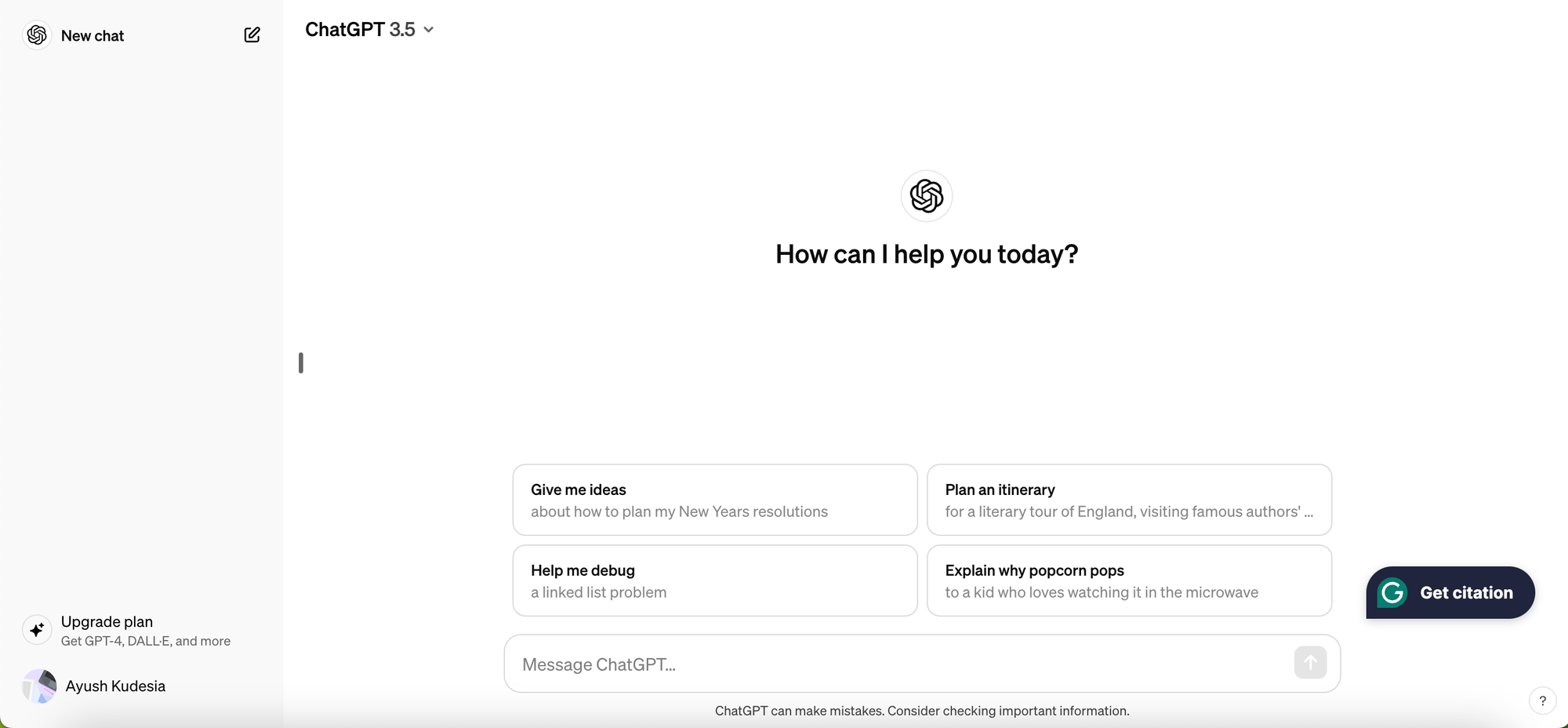This image depicts a computer screen displaying the ChatGPT interface. The background of the screen is predominantly white. In the upper left-hand corner, there is the ChatGPT logo, which is a monochrome, rope-like twisted circle. Next to the logo, the text reads "New chat." Just slightly to the right of this text is a small, square-shaped "Edit" button.

Continuing down the column on the left side of the page, there is a stardust icon next to the text "Upgrade plan," which encourages users to "Get ChatGPT for DALL-E and more." Below this, there is a thumbnail image and the name "Ayush Kudusha."

The central portion of the screen prominently displays the text "ChatGPT 3.5" with a downward arrow next to it, indicating a dropdown menu or option selection. In the middle of the page is the ChatGPT logo once more, accompanied by the greeting, "How can I help you?"

Beneath the greeting, there are several interactive boxes with text prompts: "Give me ideas," "Plan an itinerary," "Help me debug," and "Explain why popcorn pops." Below these prompts, there is a space designated for users to enter their messages to ChatGPT.

On the right side of this input area, there is a black, oval-shaped button featuring the letter "G" and the text "Get citation," suggesting a function to retrieve citations.